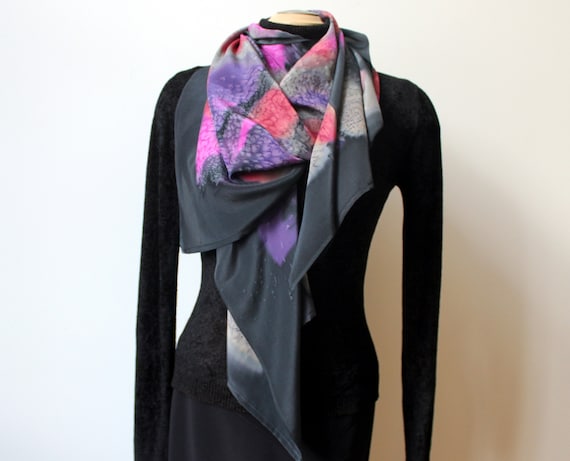The photograph features a headless and armless mannequin positioned against a solid white painted wall, occupying a square frame. The mannequin is adorned with a long-sleeved black dress, although the bottom portion of the dress is cut off and not visible within the frame. Draped casually over the mannequin's neck is a black silk scarf, decorated with an intricate pattern of purple, red, and white shapes. The scarf hangs loosely down towards where the waist would be on the dress. The mannequin's head is represented by a metallic cap at the top of its neck. There is a slight shading on the right side of the wall, potentially due to lighting in the room. The overall composition highlights the black attire and colorful scarf, creating a striking contrast against the minimalist background.